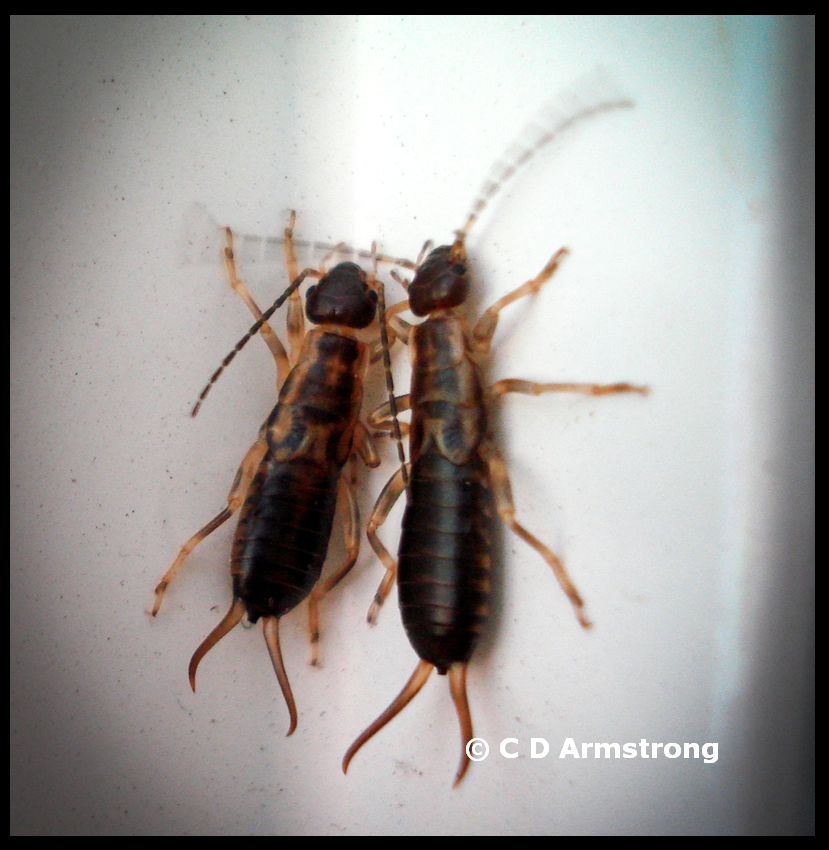The photograph, attributed to C.D. Armstrong, features a pair of black and brown cockroaches centrally positioned within a large square frame with a black border. The image is marked with a white copyright symbol and "C.D. Armstrong" in the lower right corner. Both insects are oriented vertically, with their heads towards the top of the frame and their legs and antennae extending downwards. The cockroaches' roundish, dark heads contrast with their intricately grooved bodies, which display a blend of brown and black hues. Their elongated antennae and spiky tails are notable, though slightly blurry. The background is a gradient blend, transitioning from a light grayish-brown on the left to a lighter, almost white area on the right, suggesting a light source. The insects' positions are such that the legs of the left cockroach overlap slightly with the body of the right one, adding depth to the composition.